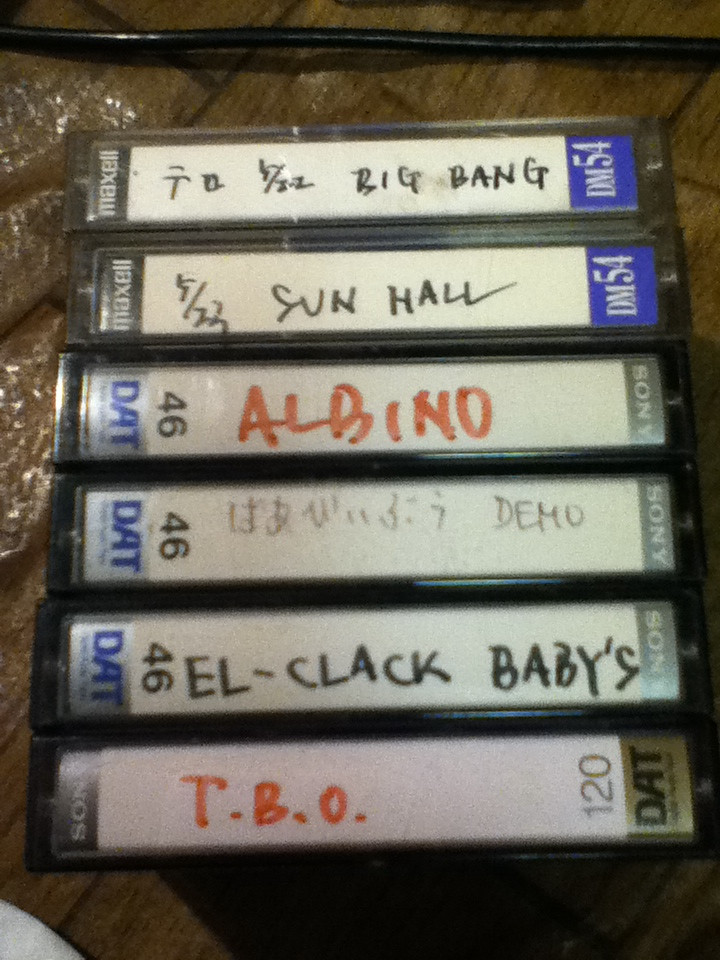The image features a stack of six cassette tapes, aligned in their glass cases and positioned with their spines facing outward. These tapes are stacked vertically on what appears to be a dark brown wooden table. Each case has a white label with handwritten text, making the labels somewhat challenging to read. From bottom to top, the first case reads "T.B.O" in red writing, the second "L Clack Babies," the third has some Japanese writing and the word "Demo," the fourth has "Albino" in red, the fifth reads "5-23 Sun Hall," and the topmost case has Japanese writing along with "5-22 Big Bang." The brands of the cassette tapes vary, with the top two cases being Maxell and the next four being Sony. A slender black wire runs horizontally across the top of the image from left to right.